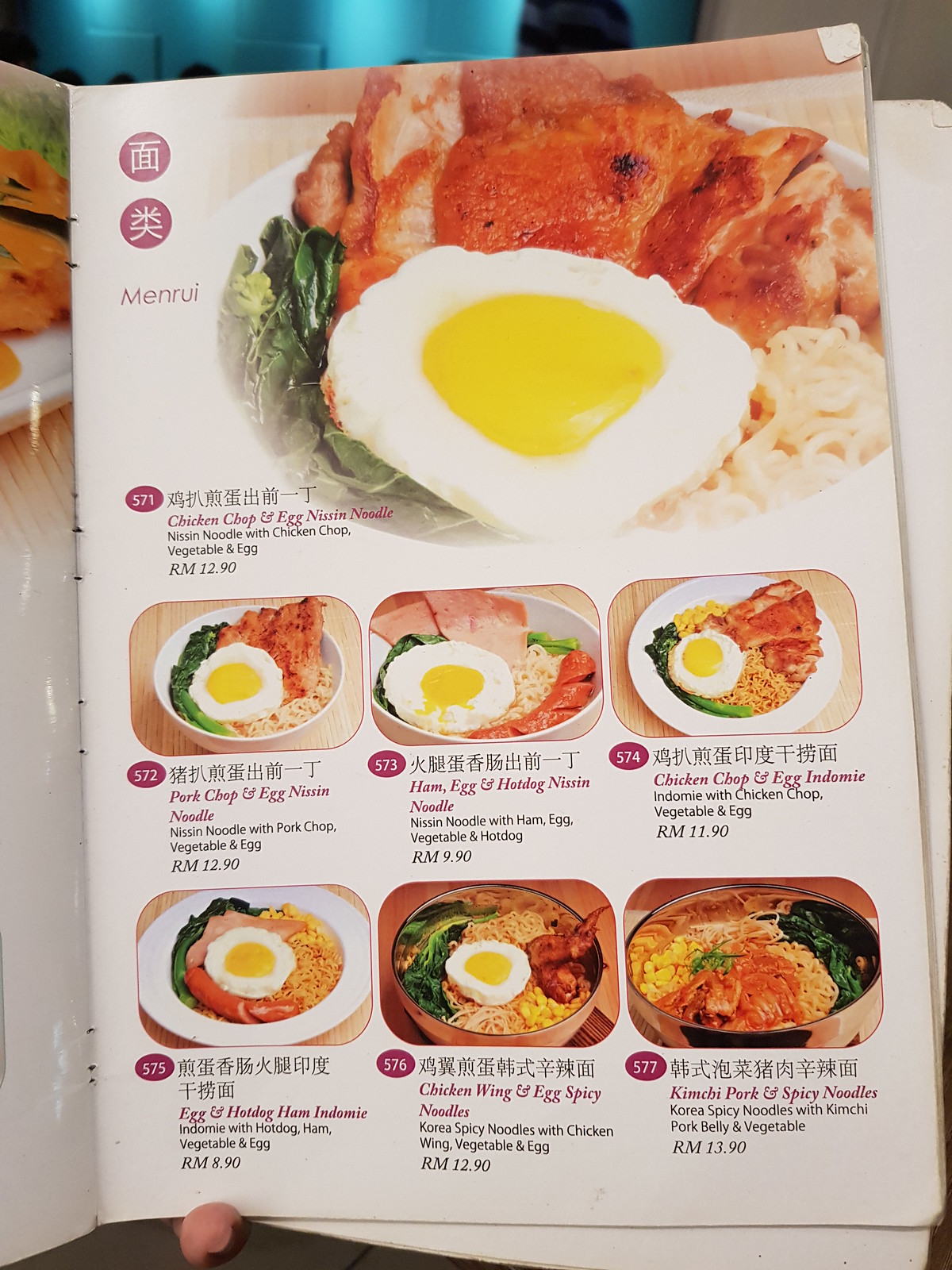This is a detailed photograph of a Japanese menu, showcasing various noodle dishes. The menu prominently features the following entrees:

1. Chicken Chop and Egg Nissin Noodles (Entree No. 571) - This is highlighted in the featured photograph at the top of the menu.
2. Pork Chop and Egg Nissin Noodles (Entree No. 572).
3. Ham, Egg, and Hot Dog Nissin Noodles (Entree No. 573).
4. Chicken Chop and Egg Indomie Noodles (Entree No. 574).
5. Egg and Hot Dog Ham Indomie Noodles (Entree No. 575).
6. Chicken Wing and Egg Spicy Noodles, referencing Korean spicy noodles (Entree No. 576).
7. Kimchi, Pork, and Spicy Noodles, also referencing Korean spicy noodles (Entree No. 577).

The menu is written in Japanese (or possibly Chinese) and includes detailed images of the dishes, showcasing ingredients like eggs, ham, noodles, and various meats. The upper left corner of the menu contains the text "MEN-RUI" along with two symbols, likely indicating a section or category of noodle dishes. The menu is open, making it easy to view all the offerings in a single glance.